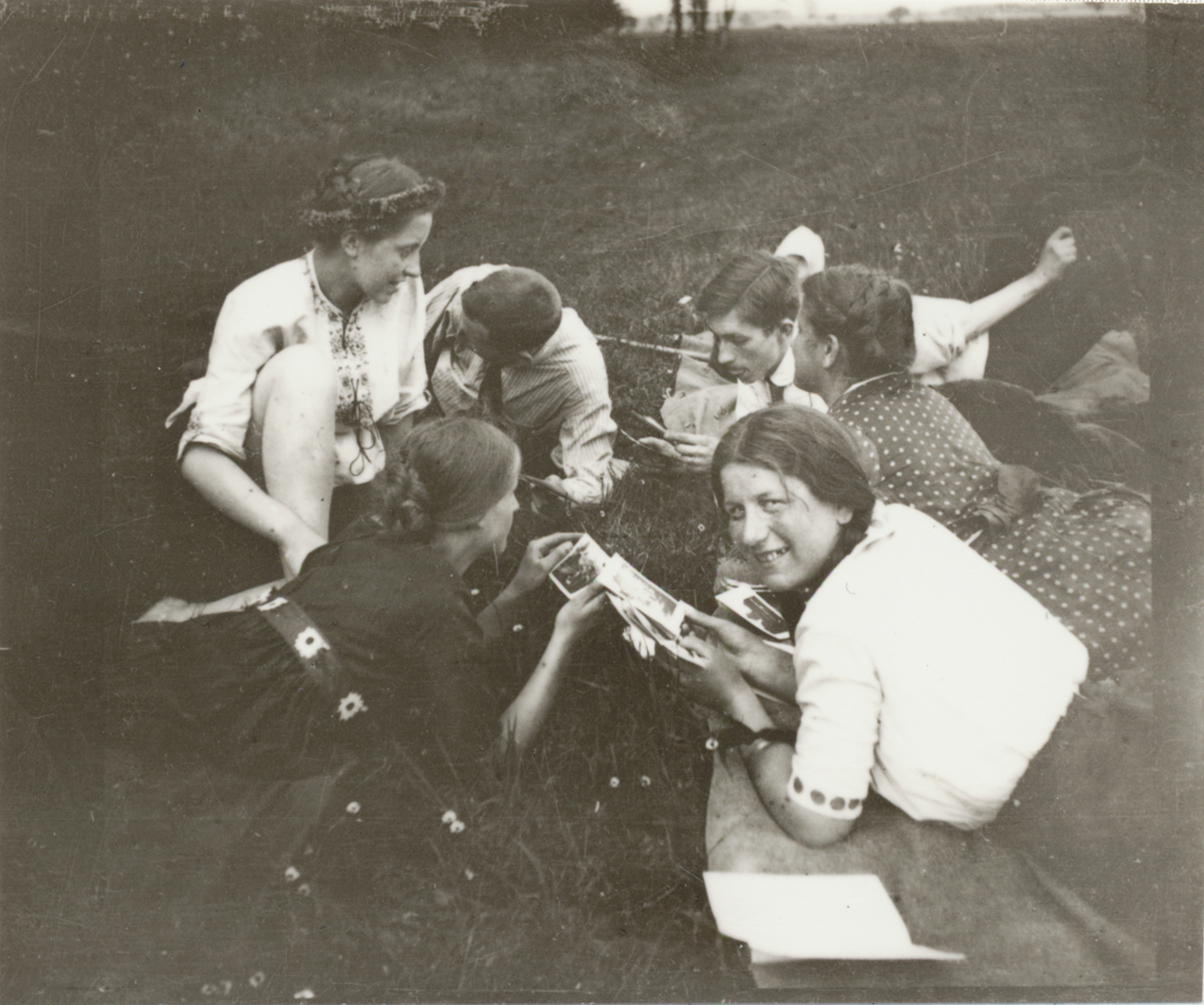This black-and-white photograph, likely taken in the 1950s or 60s, depicts a group of six people—a mix of three men and three women—relaxing in a large countryside field during daytime. The individuals are positioned close together, some seated and others lying on the grass. Prominently, there's a woman with braided hair wearing a white shirt, who is gazing over her shoulder at the camera while holding what appears to be photographs. Beside her, a woman in a polka-dotted dress observes the group. On the other side, a young man in a white button-up shirt crouches down, engrossed in the grass, while another young man in a similar white shirt looks back behind him. Additionally, there is a young woman in a white sweater with a braided hairstyle, and another woman lying on her stomach in a dark long-sleeved dress adorned with a flowered belt. The scene captures a moment of quiet interaction and contemplation, underscored by the timeless quality of the black-and-white photography.